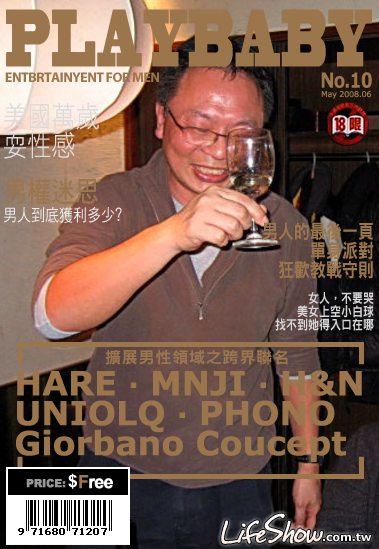The image is a tall rectangular photograph designed to mimic a magazine cover. The magazine cover is titled "Play Baby" in bold, brown block letters, accompanied by the tagline "ENTERTAINMENT FOR MEN" beneath it. Below this text, the magazine is marked as "Number 10, May 2008 06," with an "18" symbol in a circle with a diagonal line through it, indicating age restriction. The cover is adorned with Chinese characters alternating between white and gold. 

The central focus of the photograph is an older Asian man, visible from the waist up. He is wearing glasses and has short, brown hair. His attire consists of a brown zip-up sweatshirt, with rolled-up sleeves, over a gray shirt. The man’s face is slightly red, and he is smiling warmly. He holds a glass with a light-colored beverage up in front of his face, as if in a toast. His skin appears glistening, suggesting a possible state of inebriation. The background includes a large white lantern located in the top left corner. At the bottom right of the cover, the website "LIFESHOW.COM.TW" is displayed. Additional details include a barcode at the bottom left, labeled "Price Free."